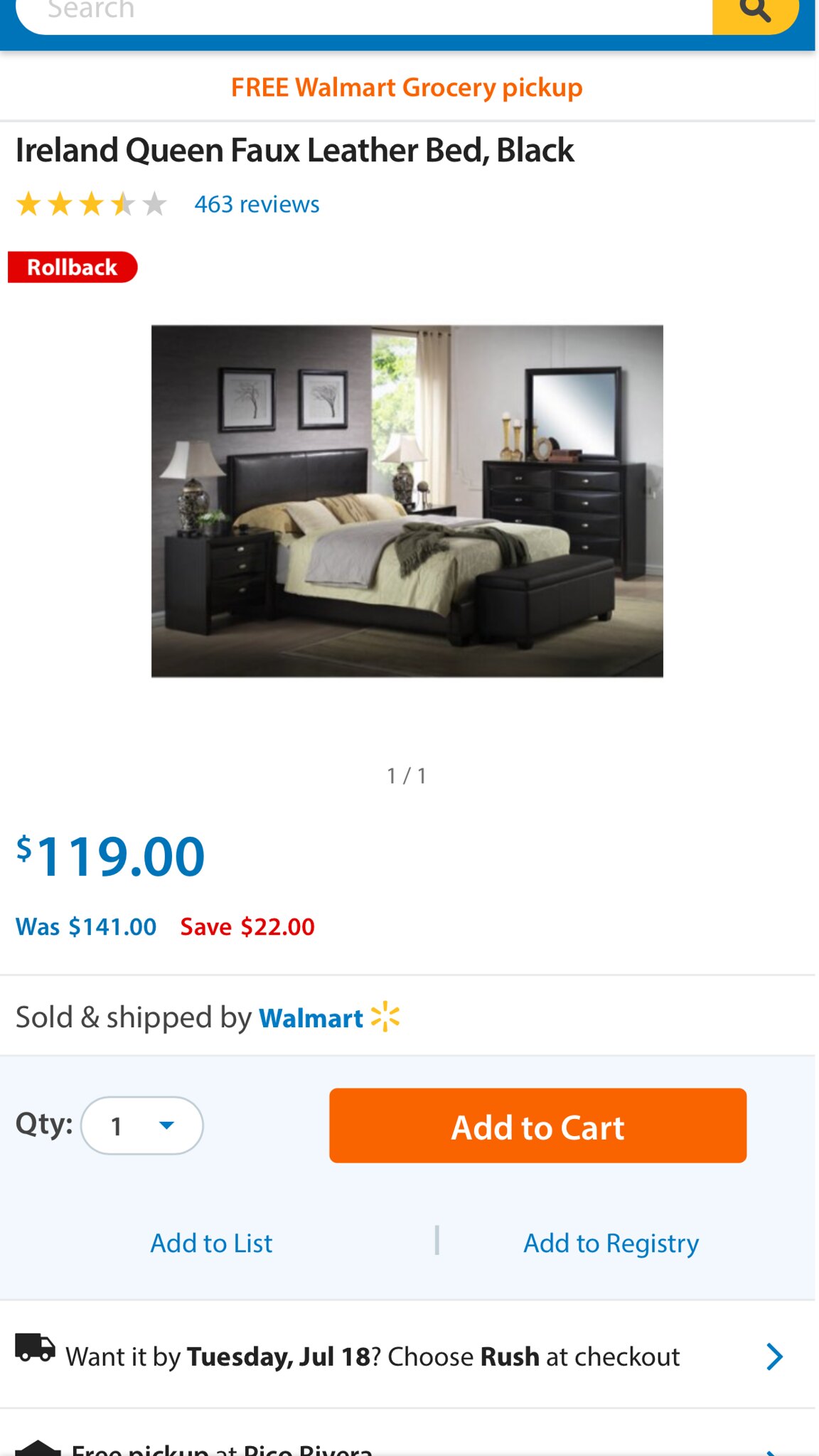This screenshot captures an advertisement listing on Walmart's website for an Ireland Queen Faux Leather Bed in black. At the top of the image, the Walmart search bar is visible, along with the text "Free Walmart Grocery Pickup." The bed has a 3.5-star average rating based on 463 reviews. Displayed in red text, the item is marked as a rollback, originally priced at $141 and now offered at $119, saving $22. The bed features a black headrest and a matching bench at the end, adorned with neatly arranged linens. It is sold and shipped by Walmart, and there's an option for expedited checkout to receive the item earlier. Additional options on the page include adding the bed to the cart, a list, or a registry. The listing also mentions the possibility of free pickup at a specific location, though the detailed text is partially cut off.